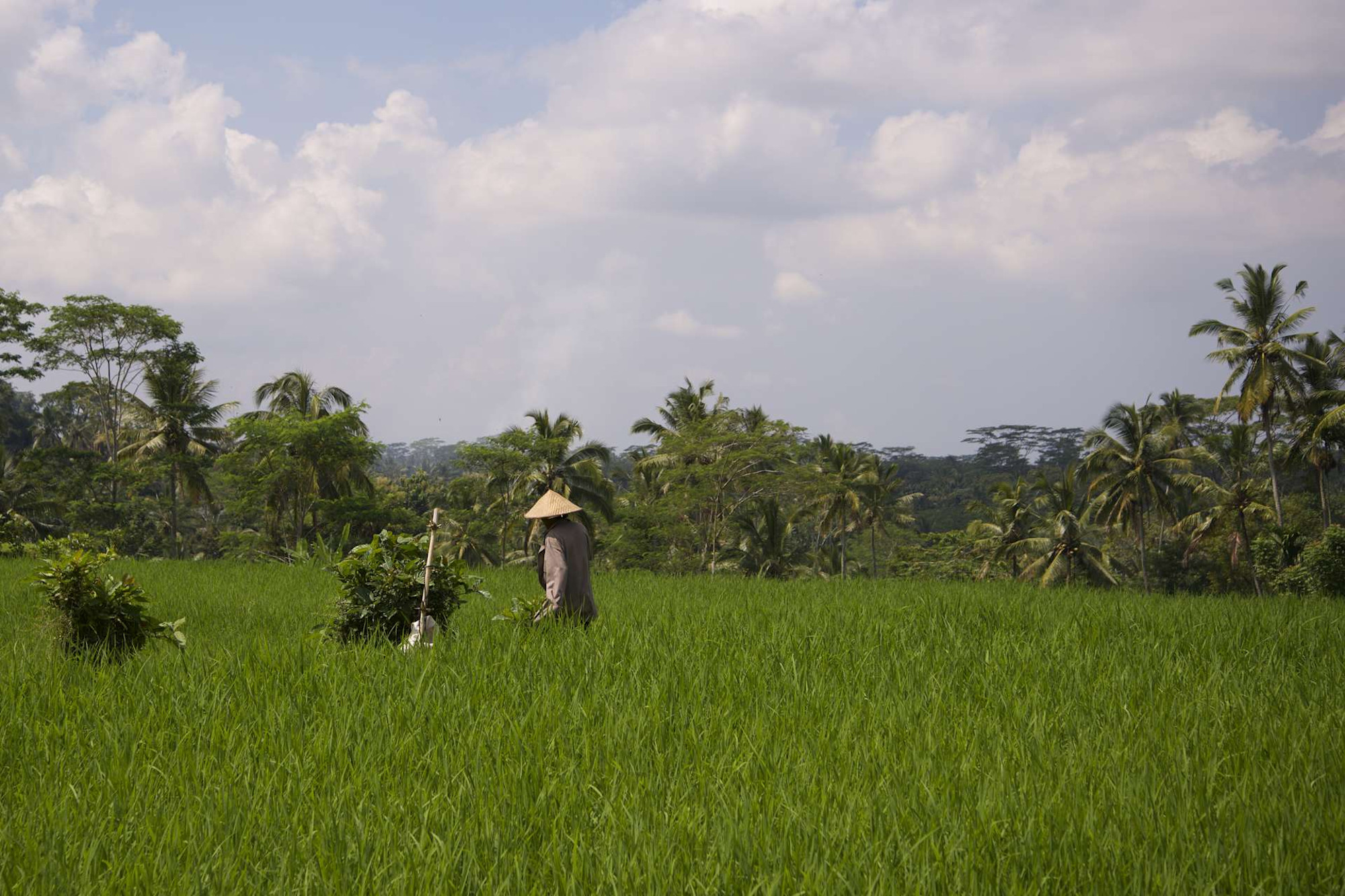In this image, we see a man standing in the middle of a lush, green field, possibly a rice field, surrounded by tall grass. The man is wearing a straw conical hat that stands out with its tan color and a long-sleeve gray garment. He is positioned slightly to the left of the center of the image. To his immediate left, a stick or shovel is leaning against a bush. The vibrant green grass dominates the foreground, extending almost to the middle of the image. In the background, a tree line composed mostly of palm trees runs from left to right, with a few other types of trees mixed in. Above this verdant scene, the sky takes up a significant portion of the image, exhibiting a light blue hue punctuated by fluffy white clouds. The overall setting appears to be tranquil and rural, possibly in an Asian country, and the image evokes themes appropriate for travel or agricultural websites, highlighting the natural beauty and simplicity of the landscape.